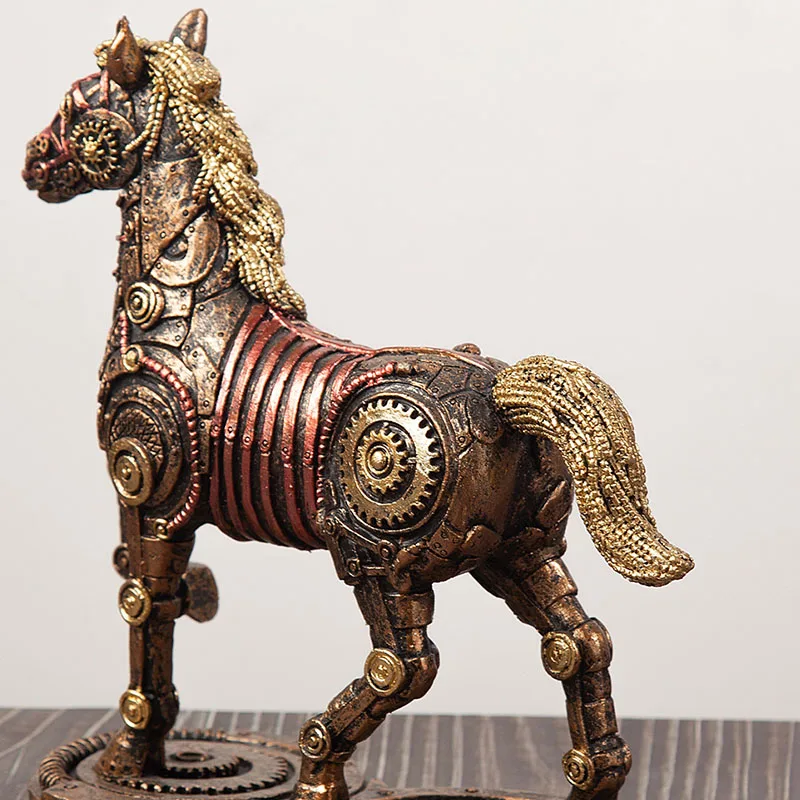This photograph showcases an intricately designed metal sculpture of a horse, embodying a steampunk aesthetic with clockwork and mechanical elements. The horse's body is composed of interlocking metal plates and gears, with rivets and wiring that emphasize its mechanical nature. Its mane and tail appear as chains or strings of metallic beads, complementing the overall detailed craftsmanship. The color palette is a rich blend of gold, brown, tan, and bronze, highlighting various parts of the horse including its golden mane, tail, and delicate ears. The sculpture stands on a base made of gears, reinforcing its steampunk design. This striking figure rests atop a dark brown tabletop with light gray striations, set against a simple white wall, which draws full attention to the horse as the focal point of the image. The meticulous detail in the metalwork and the lifelike yet fantastical design of the horse create a captivating and detailed visual experience.